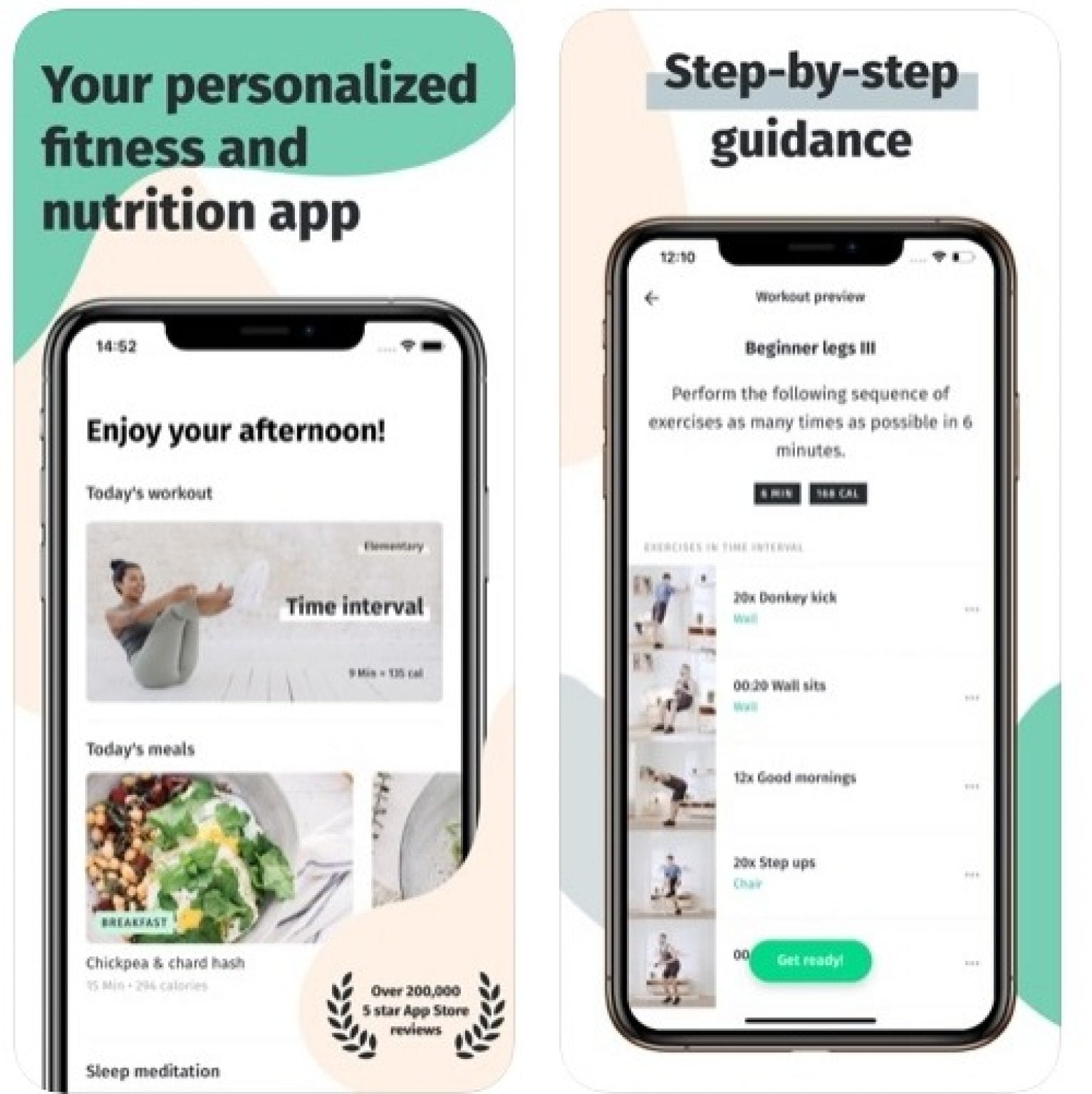In this advertisement, two smartphones are displayed side by side, showcasing a fitness and nutrition app. The smartphone on the left prominently features the bold title "Your Personalized Fitness and Nutrition App" at the top. Its screen displays an image of a woman performing sit-ups or crunches, symbolizing physical exercise. Below this, there is a picture of a healthy dish consisting of chickpeas and salad, emphasizing nutrition. Furthermore, an award stamp highlighting "Over 200,000 Five Star App Store Reviews" is also visible on this screen, underscoring the app's popularity and credibility.

The smartphone on the right is shown with a list of exercise videos, emphasizing practical workout routines. The title at the top of this phone reads "Step-by-Step Guidance," indicating the app's focus on providing detailed instructions. Both images collectively suggest a comprehensive approach to fitness and healthy eating. The overall presentation clearly aims to advertise a comprehensive fitness app designed to assist users in achieving their health and fitness goals through personalized exercise and nutrition plans.